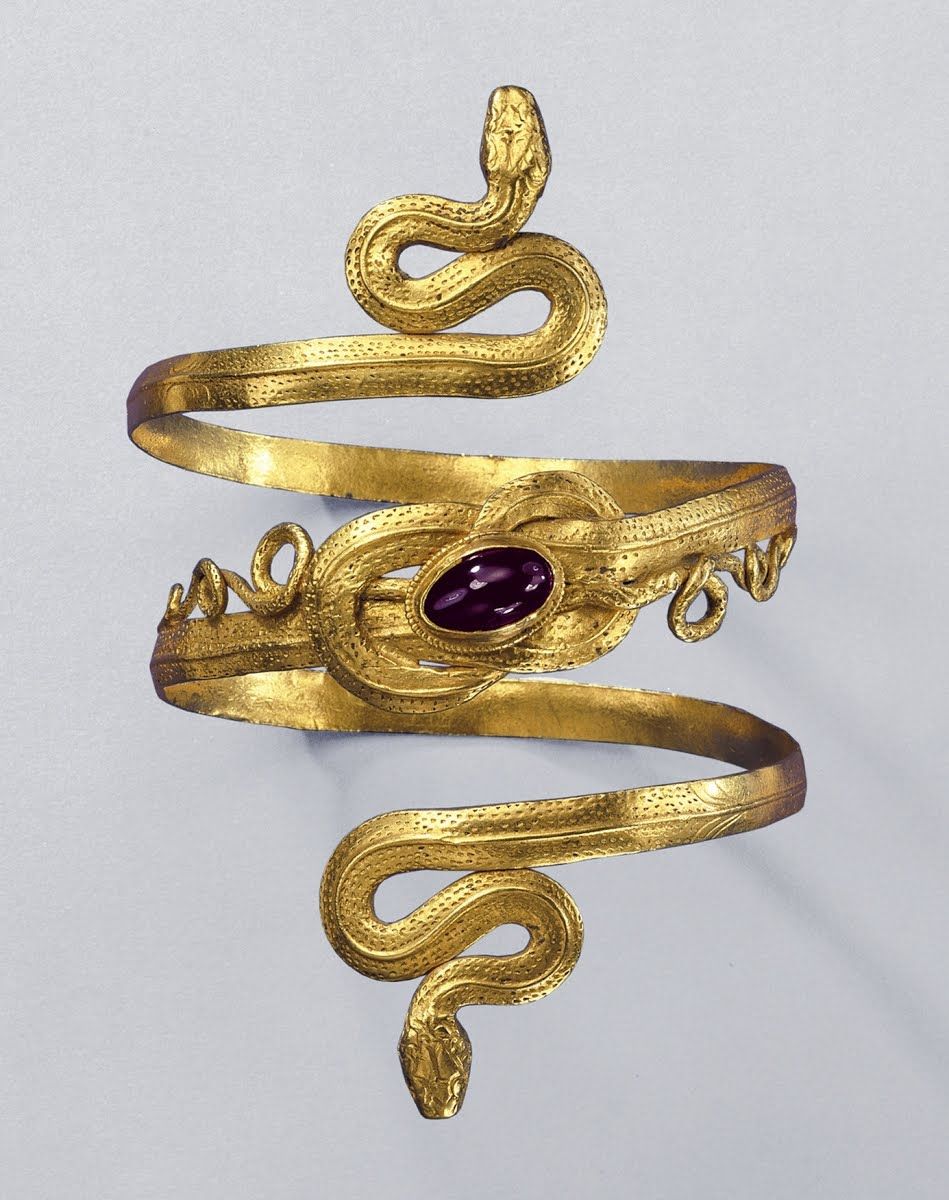This photograph captures a detailed arm or wrist wrap bracelet, presented as the sole object against an off-white, light gray background. The bracelet is crafted from a gold-colored metal and intricately designed to represent two entwined snakes. Each end of the bracelet features a snake head, with their bodies forming elegant, sinuous curves that wrap around, resembling an "S" shape. The tails of the snakes converge at the center, where a prominent, oval-shaped gemstone is embedded within the gold. This jewel, appearing as a mix of dark brownish and purplish hues, is encircled by elaborate metalwork, adding to the bracelet’s ornate and sophisticated design. The meticulous craftsmanship on the snakes’ scales and the overall intricate details highlight the bracelet's elegance and fine artistry.